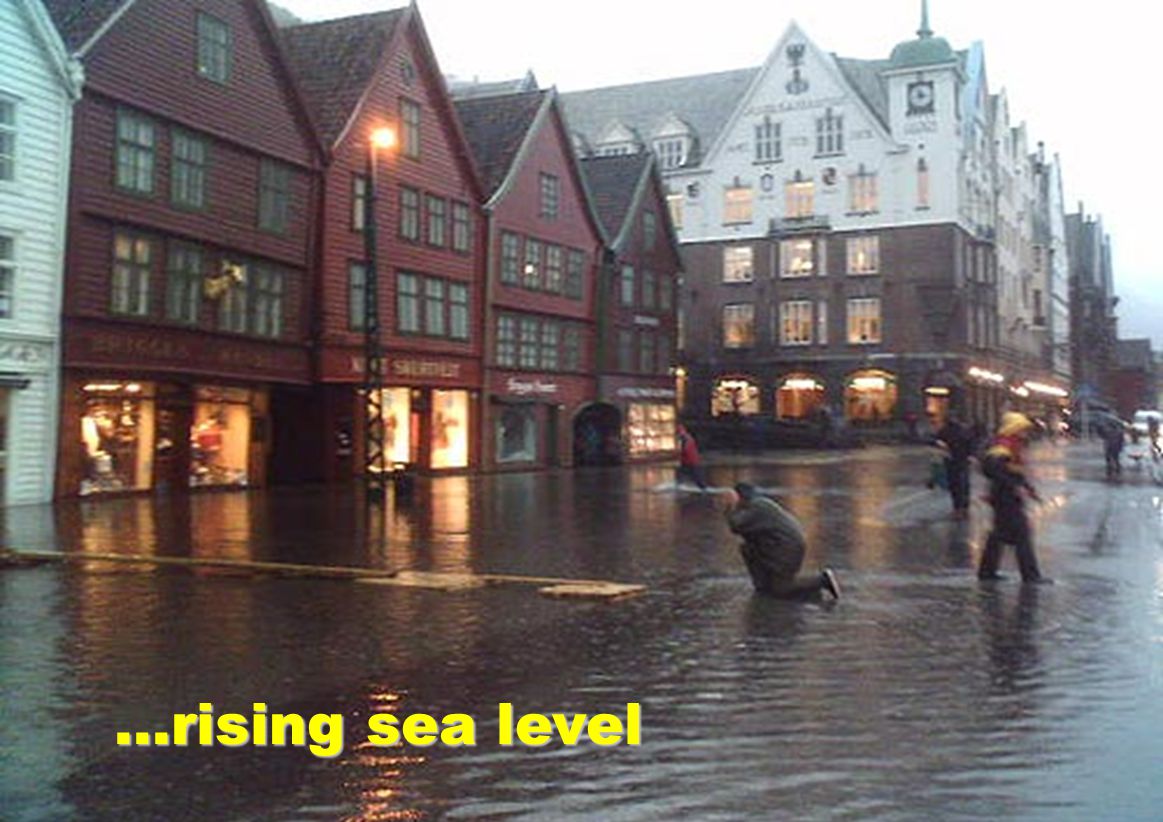The image depicts a small town street that is flooded, with a man kneeling in the water in the foreground, causing ripples to radiate around him. The street is submerged, with no visible dry ground, indicating heavy rainfall. On the left side of the street, there is a row of four dark red buildings, all identical in shape and window arrangement. In the background, a larger building stands higher than the red ones, with a distinctive triangle-shaped white top, nine windows arranged in two at the peak, three below the triangle, and three in two rows on the brown bottom half. The bottom of this larger building is lit up, showcasing three illuminated archways. At the bottom left corner of the image, in bright yellow text, are three dots followed by the words "rising sea level." There are various people walking through the flooded street, and it appears to be still lightly raining.